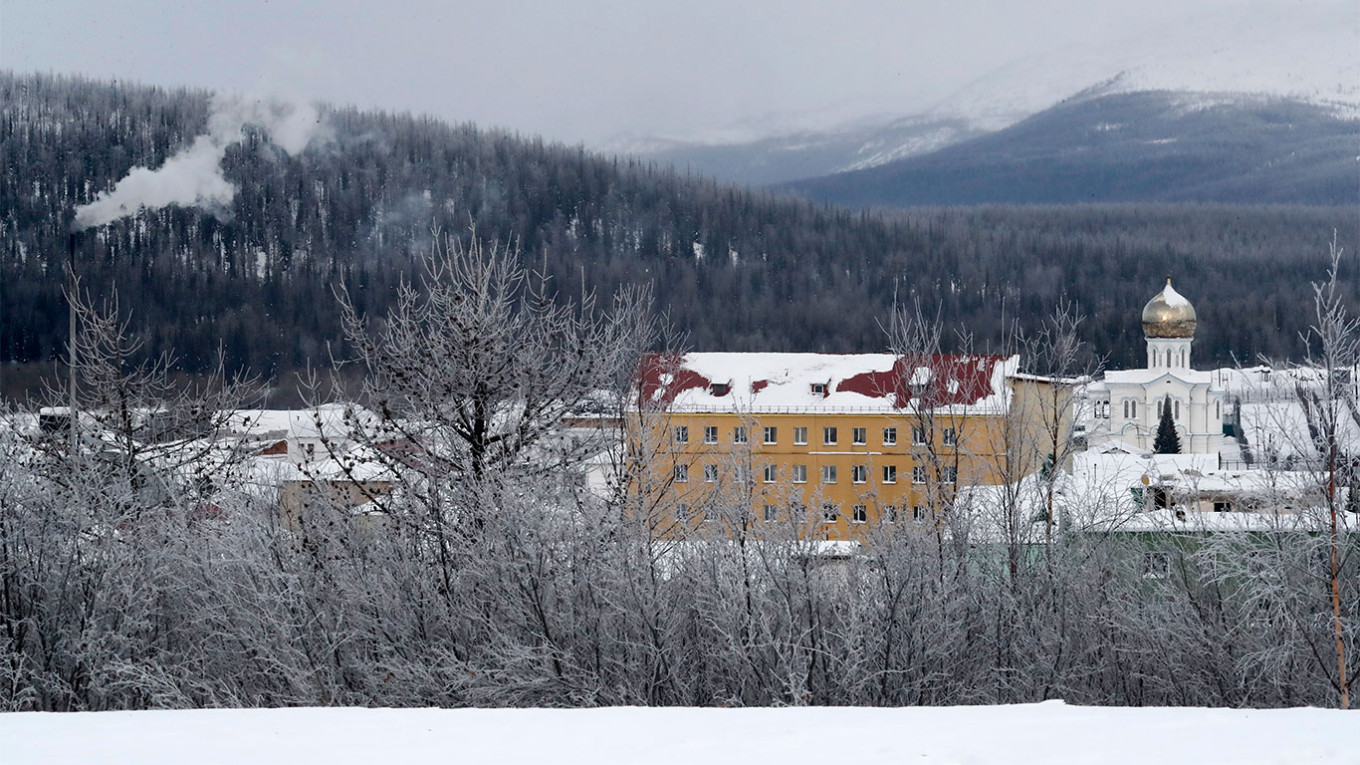The photograph captures a picturesque, snowy landscape with remarkable detail. At the center of the image, there is a cluster of large buildings, suggesting a small city or village scene nestled amidst a substantial evergreen forest. Prominent among these structures is a three-story orange building capped with a dark red roof, partly blanketed in snow. Close by stands a striking white building crowned with a gold dome, evoking the architecture of a mosque or church. The scene also features bare trees in the foreground, their branches cloaked in snow. The background is dominated by majestic mountains with snow-covered peaks, beneath a sky streaked with varying shades of gray clouds. The fading hues of the sky and the serene snow-covered field enhance the ethereal quality of the image, creating a tranquil winter scene.